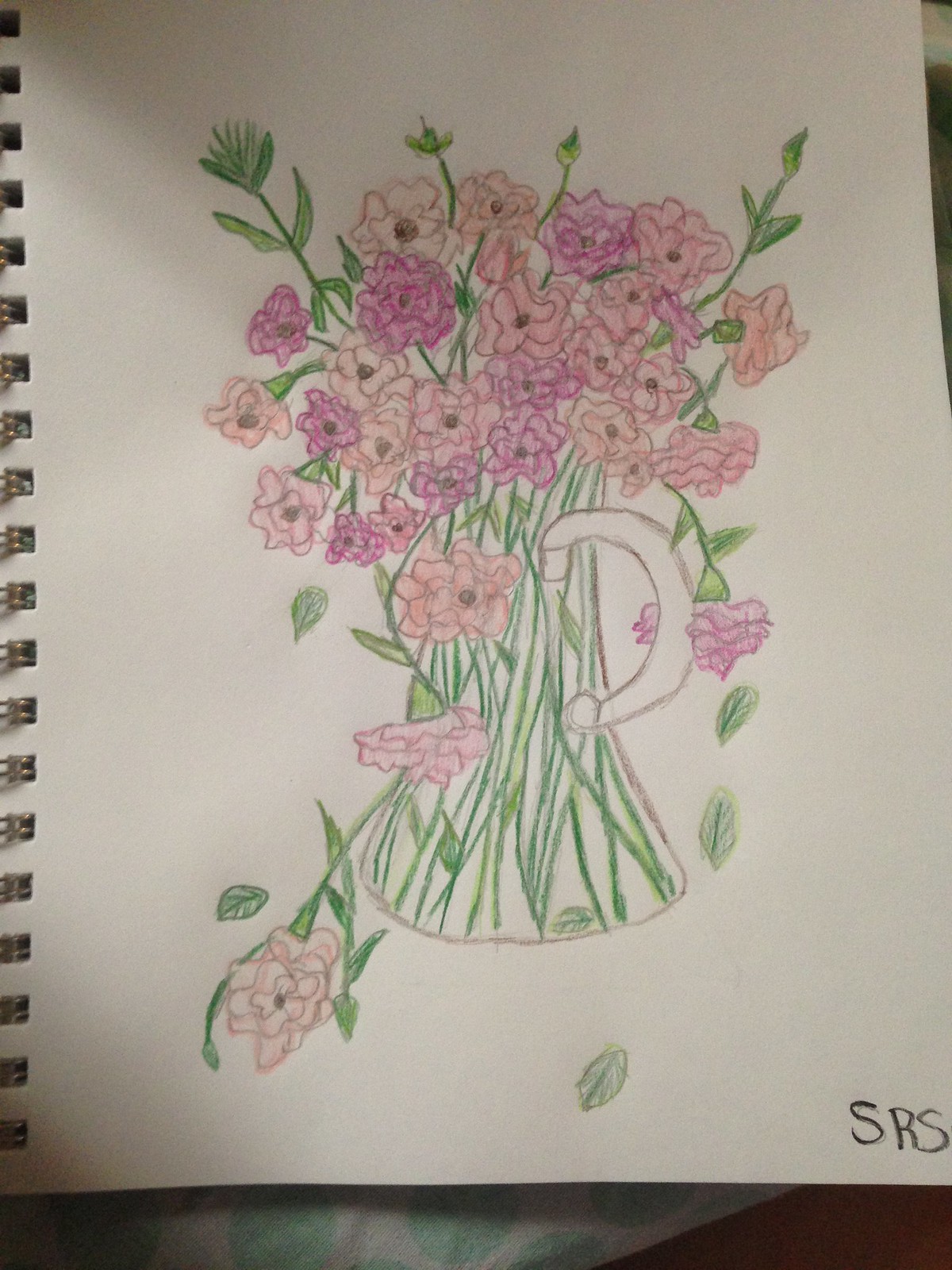The photograph captures a detailed drawing on a page from an art notebook, which is placed on a surface adorned with a white fabric featuring green polka dots. The notebook reveals spiral binding on the left side, and the bottom right corner of the page is marked with the initials 'SRS,' presumably identifying the artist. The drawing itself depicts a clear glass vase, outlined in black to indicate its transparency, with a wide bottom narrowing at the top, and a handle sketched in pencil without shading. Inside the vase, we see green stems conforming to its shape, suggesting a collection of flowers in the vase. The flowers are a mix of light pink, dark pink, and purple hues, resembling carnations. Some of the flowers hang downwards while others stand upright, surrounded by shoots and green leaves, adding to the overall lushness of the arrangement. The artistry, marked by its simplicity, suggests that it might have been created by a young artist, possibly a child or teenager.